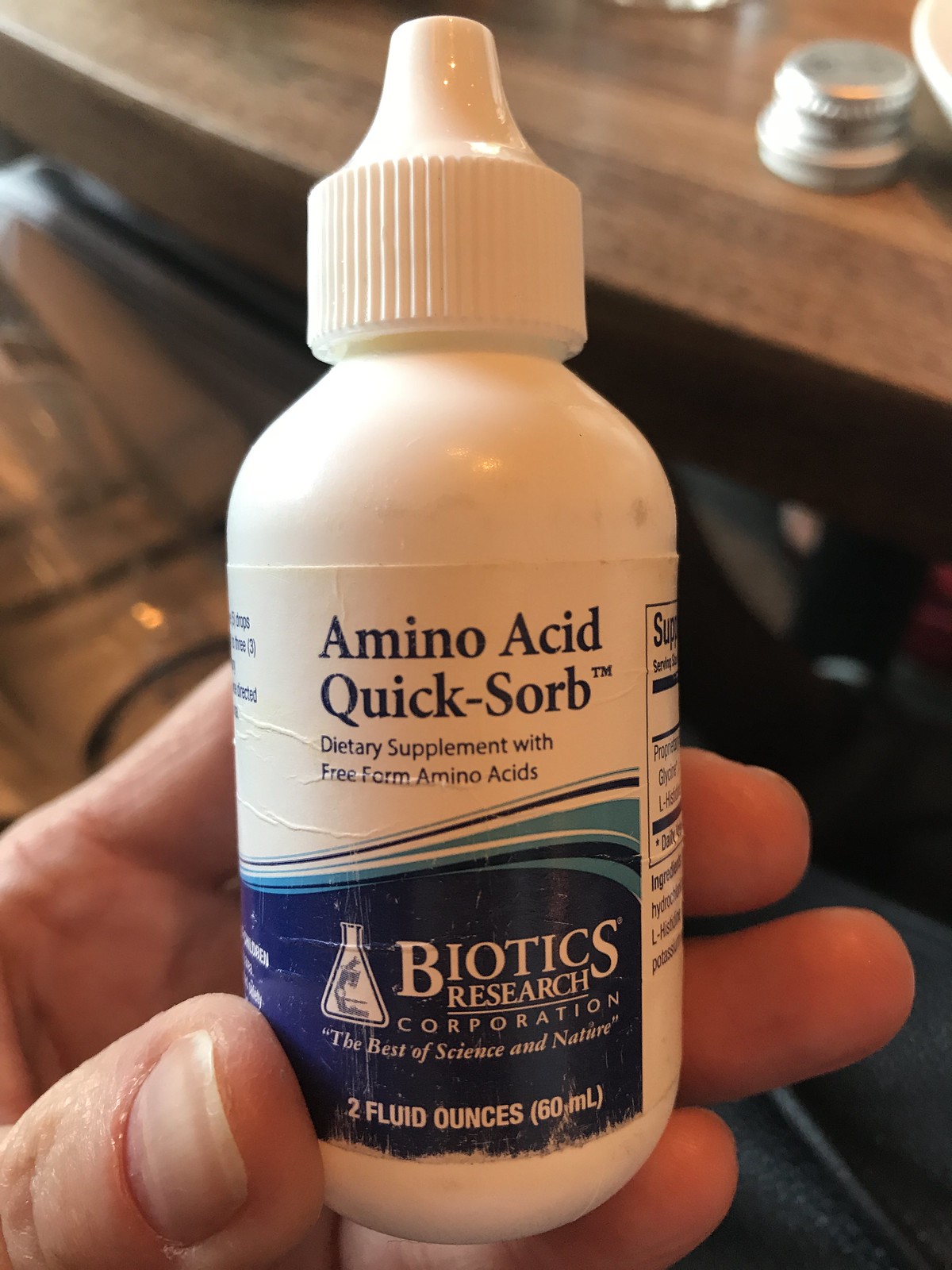A detailed photograph showcases a hand holding a small white bottle of a dietary supplement. The person holding the bottle has very light skin and clean nails. The bottle prominently displays the label "Amino Acid Quixorb Dietary Supplement with Free Form Amino Acids." It also mentions "Biotics Research Corporation, the best of science and nature." The label is primarily white with a blue lower half. At the bottom of the label, the volume is specified as "2 fluid ounces (60 ml)."